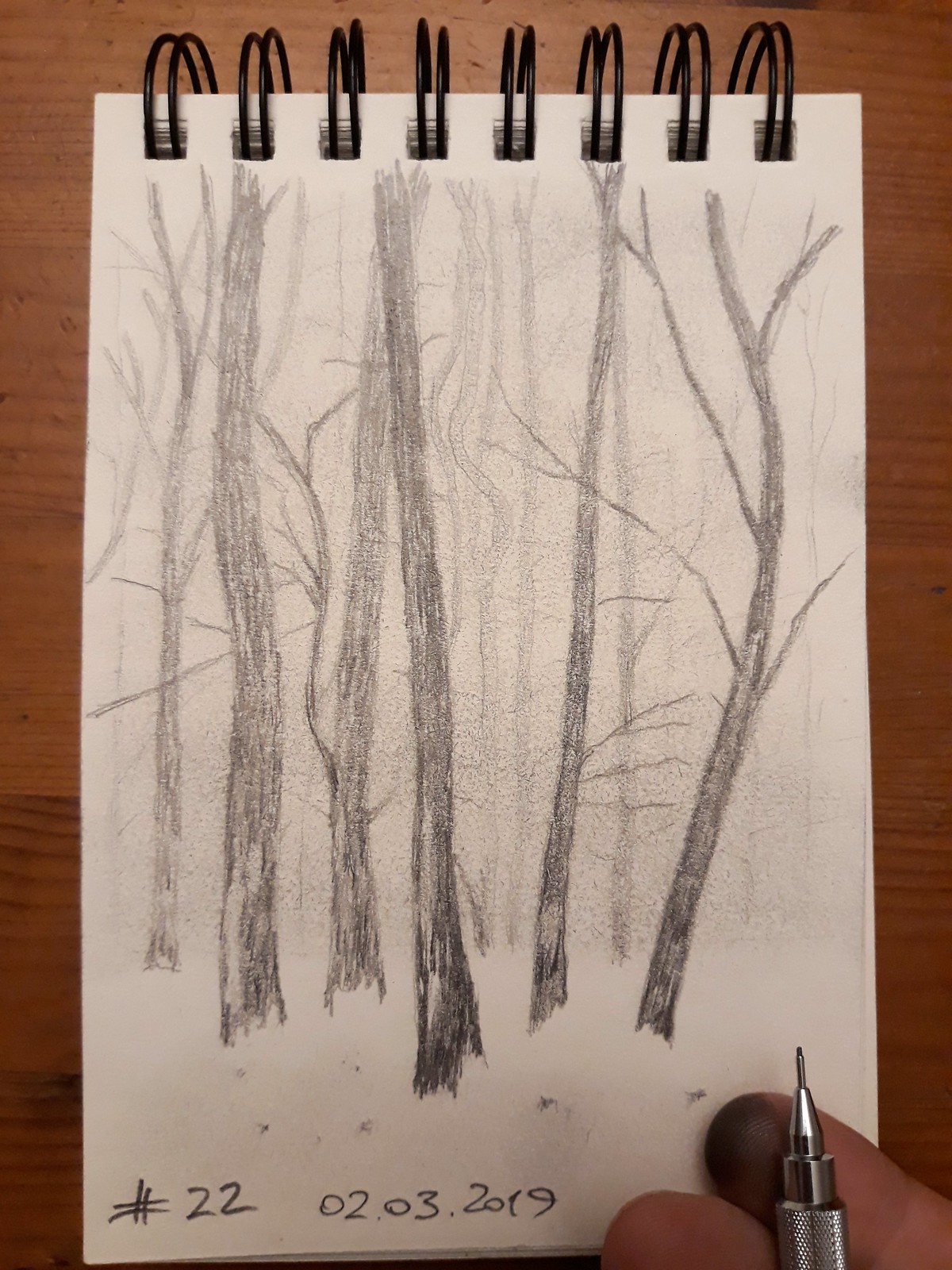A detailed graphite pencil drawing of a serene winter forest scene is meticulously rendered on a white, spiral-bound sketch pad resting vertically on a wooden tabletop. The artwork features a series of bare tree trunks and branches, with the bottom section left unshaded to evoke the presence of snow. The date "22-02-03-2019" is inscribed by the artist on the drawing, while the tip of a mechanical pencil is also visible, held by the artist, conveying the painstaking craftsmanship involved.